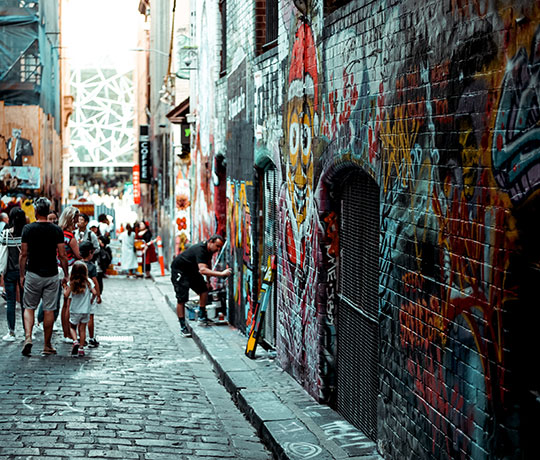The photograph, taken outdoors during the daytime, captures a bustling, narrow alleyway or walkway from an aerial perspective. The ground on the left-hand side is lined with brick paver stones, painted a light gray, adding a subtle texture to the scene. Numerous people, dressed in summer attire such as shorts and t-shirts, are casually strolling down the street, adding a lively atmosphere.

Dominating the center of the image is a raised ledge leading to a large brick wall that extends upward, creating a boundary on the left. This brick wall, adorned with various graffiti, features several arched doorways embedded within it, adding architectural interest. In the midst of the vibrant street life, a man with light brown skin, dressed in a black short-sleeved t-shirt and black shorts, is seen painting the graffiti-covered wall. Despite his artistic endeavor, the passersby seem unperturbed, absorbed in their own activities. The entire scene exudes a blend of urban grit and communal energy, encapsulating the essence of street life.